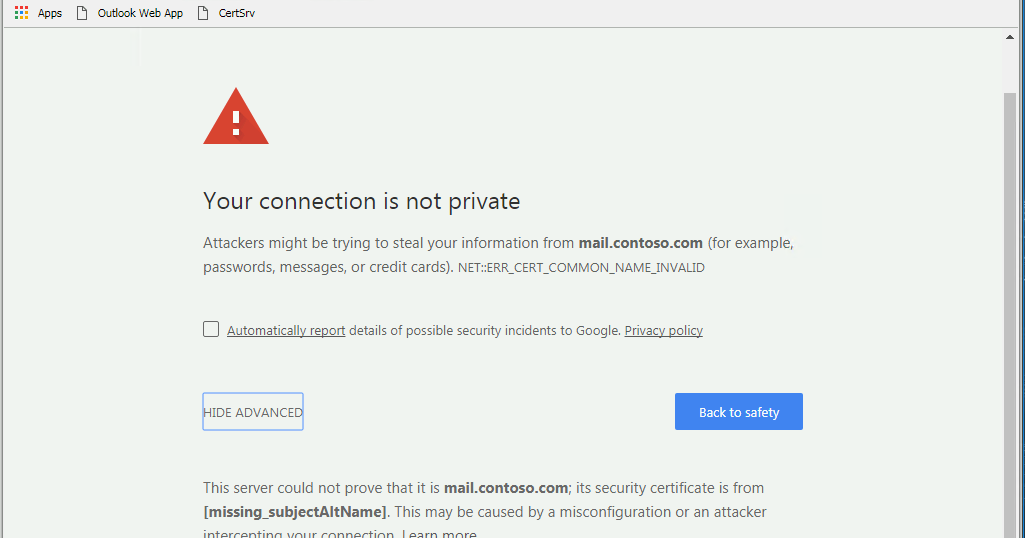This image showcases a security alert within a web browser, detailing that the connection to the site is not private. 

At the upper left corner, there is an array of app icons arranged in a 3 by 3 grid pattern, each dot representing various apps in different colors. Adjacent to these icons, there is a dog-eared page icon symbolizing the Outlook Web App, followed by another icon for CertSRV.

Dominating the main area of the image is a red triangle with a drop shadowed exclamation mark inside it, indicating a warning. The prominent text within the alert reads, "Your connection is not private," cautioning that attackers might be attempting to steal information from `mail.contasso.com`, such as passwords, messages, or credit card details. The specific error displayed is "NET::ERR_CERT_COMMON_NAME_INVALID," with underscores separating each word.

Below the warning message is an unchecked checkbox labeled "Automatically report details of possible security incidents to Google," accompanied by an underlined text link titled "Privacy policy." 

Further details are enclosed within a blue-rectangular border, which may either signify a button or simply enclose the text in a tightly packed manner. The blue button to the right is labeled "Back to safety," providing an immediate action for the user to retreat from the unsafe connection.

At the bottom, partially cut off by the edge of the image, there is an additional message stating, "This server cannot prove that it is `mail.contasso.com`; its security certificate is from `MISSING_SUBJECT_ALT_NAME`." It suggests that this issue may be due to a misconfiguration or an attacker's interception of the connection. The final line of text, beginning with "Learn more," is truncated, showing only the top half of the words.